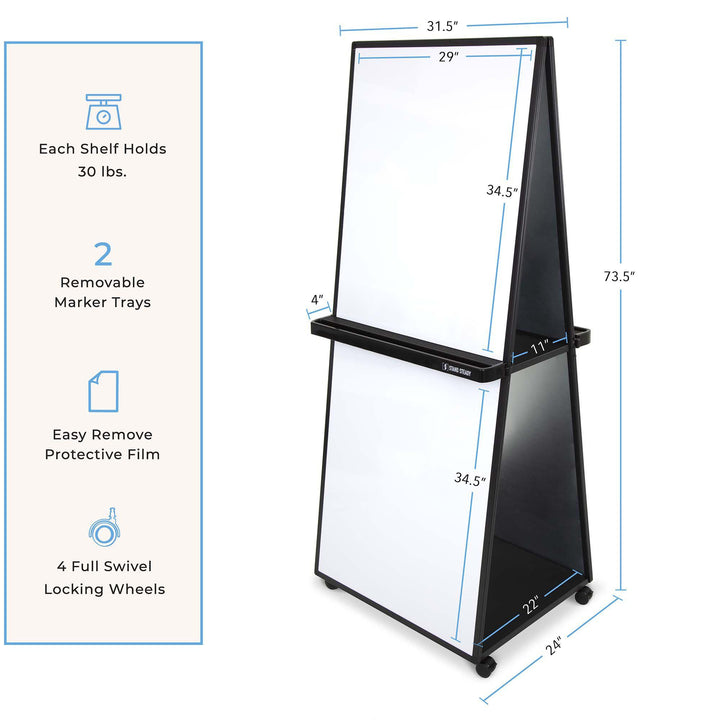This detailed diagram showcases a versatile artist's easel designed in an A-frame structure with dual boards, making it an ideal tool for creative activities. The easel stands 73.5 inches tall and features a base width of 24 inches, allowing stable mobility on four swivel-locking casters. The front section, with a light pink background and blue border, measures 29 inches wide by 34.5 inches tall, providing ample space for writing or drawing. The whiteboard area is split by a 4-inch deep tray, perfect for holding markers and other supplies. The back section mirrors the front, supporting the A-frame structure, and includes a second marker tray. 

The detailed diagram includes important specifications: Each shelf can support up to 30 pounds, the trays are removable, and the protective film is easily removable. The black casters ensure the easel can be securely positioned and moved as required. The left side of the diagram breaks down these features with corresponding visual icons in blue, enhancing usability for children’s rooms or creative spaces, making it a practical and engaging tool for artistic endeavors.